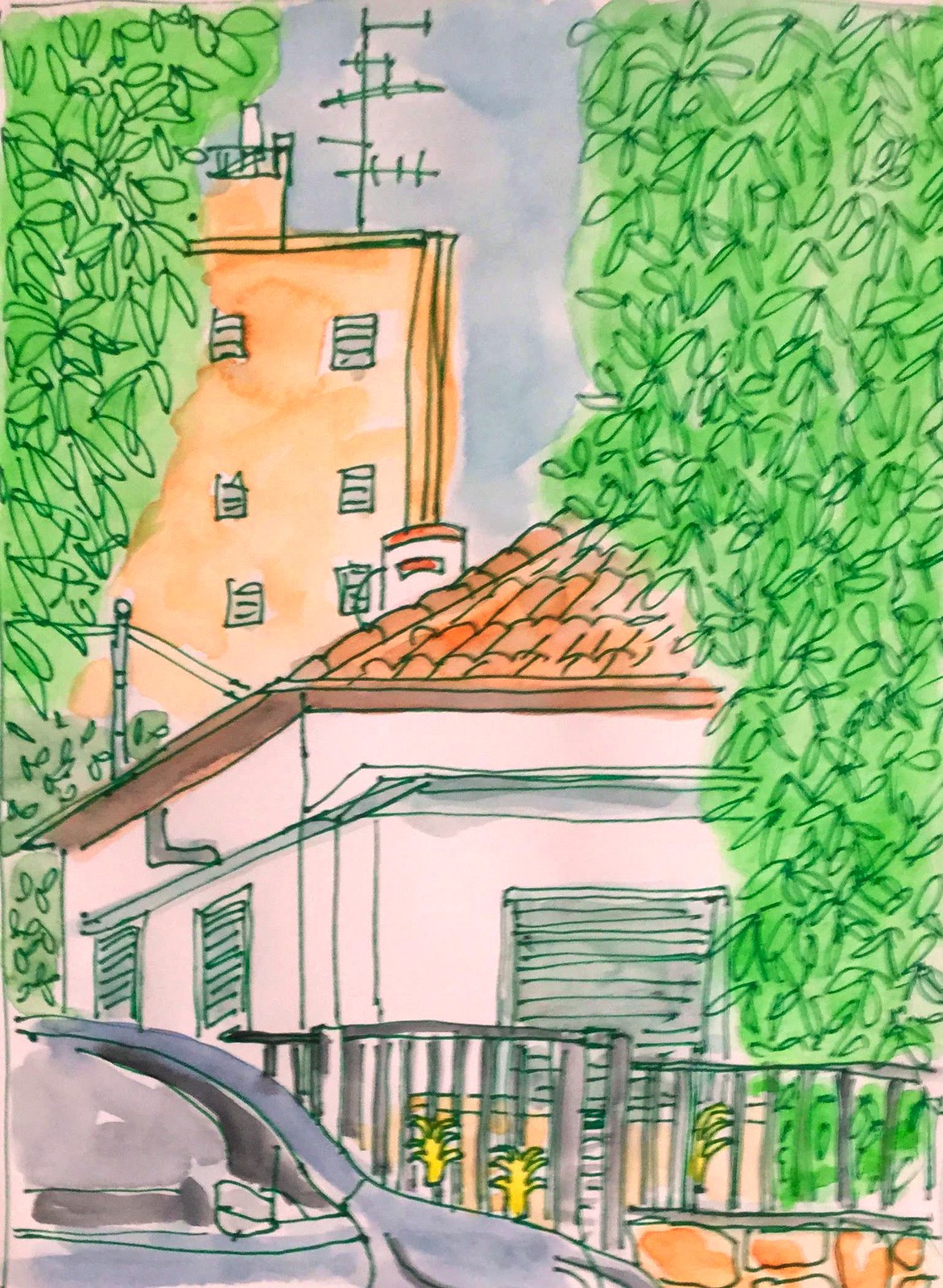This detailed colored drawing captures a vibrant street view showcasing a cartoonish-style, slightly distorted perspective devoid of straight lines. On the bottom left corner, a gray sedan marks the foreground, characterized by gray-tinted windows. Positioned behind the car is a silver metal fence featuring a vertical post. Beyond this fence stands a quaint, single-story white house adorned with bluish-gray shutters. The house is topped with a staccato roof composed of reddish-brown, overlapping tiles. Lush green shrubbery flanks the house on both sides, adding to the richness of the scenery. In the background, a tall brown apartment building with smooth sides and gray windows rises, sporting an antenna on its rooftop. Completing the scene, a bluish-gray sky stretches above, lending an open-air feel to the artwork.